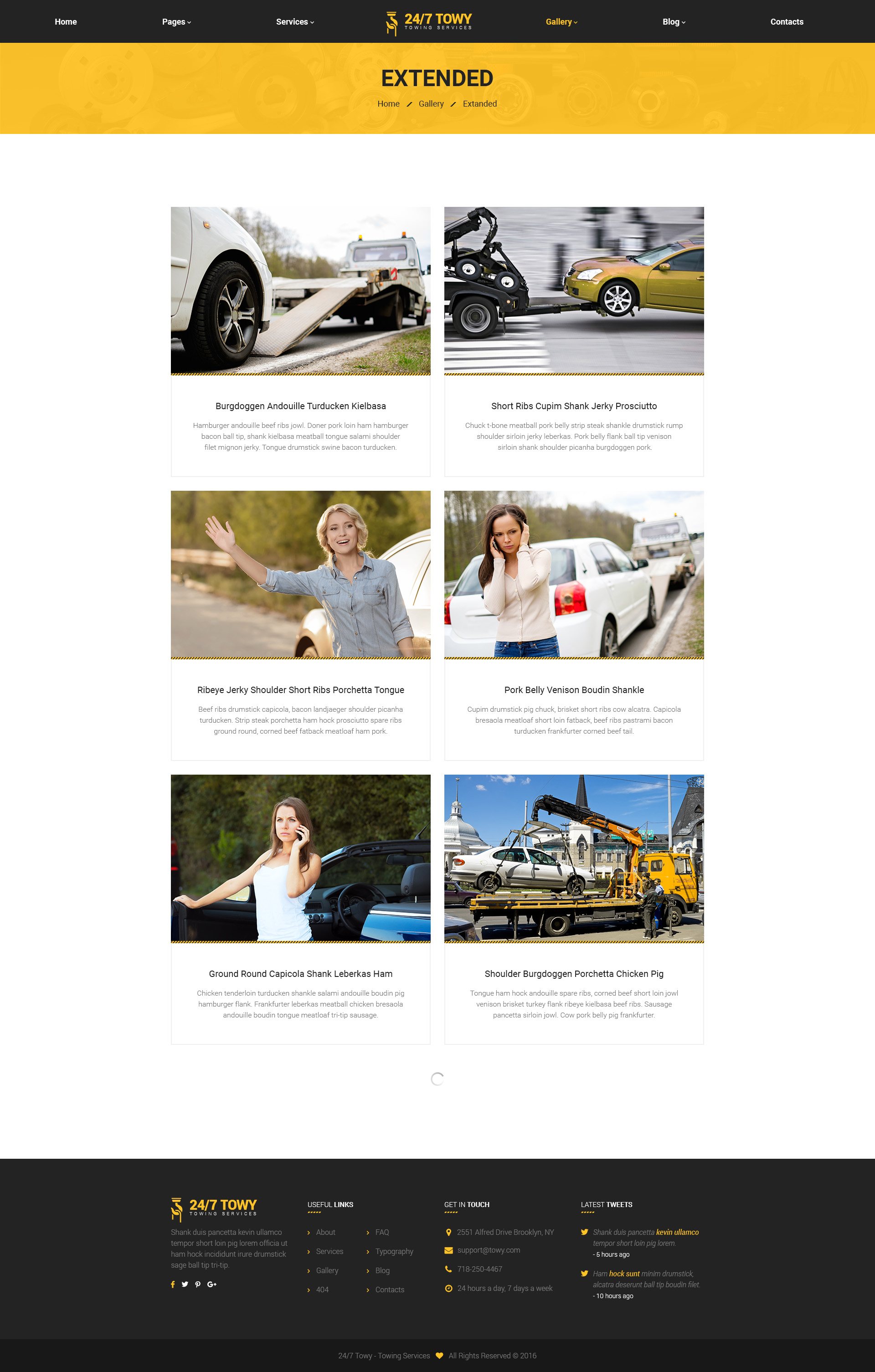Here is a refined and detailed caption for the described image:

---

This web page from 24-7 TOWV features a sleek and structured design. The page is vertically rectangular, framed by thin black ribbons at the very top and bottom of the screen. The top black ribbon showcases navigational text in white, listing 'Home,' 'Pages,' 'Services,' 'Gallery,' 'Blog,' and 'Contact' from left to right, with 'Gallery' highlighted in gold. Centered within this ribbon is the business name, "24-7 TOWV," accompanied by its gold logo to the left.

Directly below the top ribbon, a thicker gold ribbon spans the width of the page, prominently displaying the word "EXTENDED" in bold black capital letters. Beneath this, on a white background, the page is organized into six distinct rectangular sections, each containing an image with a black-text caption underneath. Below each caption is a brief description in light gray text, providing further details about the images.

At the bottom of the page, a wide dark gray banner stretches across the screen, filled with various content options, including help, contact information, and links to different services. Additionally, this banner features icons for connecting to social media platforms.

---